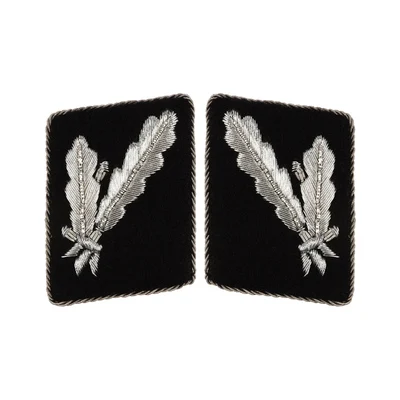The image showcases two identical badges or patches set against a stark white background. Each patch is a black square meticulously adorned with three embroidered silver leaves, set in a mirrored arrangement. The central leaves feature intricate claw-like talons at their base, all unified by a silver thread that binds them together. Both badges are bordered by a silver-stitched edge, resembling a gray rope. The embroidery is detailed, with varying shades of gray used to indicate depth and texture within the feathers, giving the appearance of light and dark gray hues. The central motif appears almost sketched, with more intense, darker areas marked by scratch-like strokes, contributing to a dynamic grayscale composition. The symmetrical presentation of the badges, angled slightly upwards toward the middle of the image, reinforces their mirrored symmetry and visual harmony.